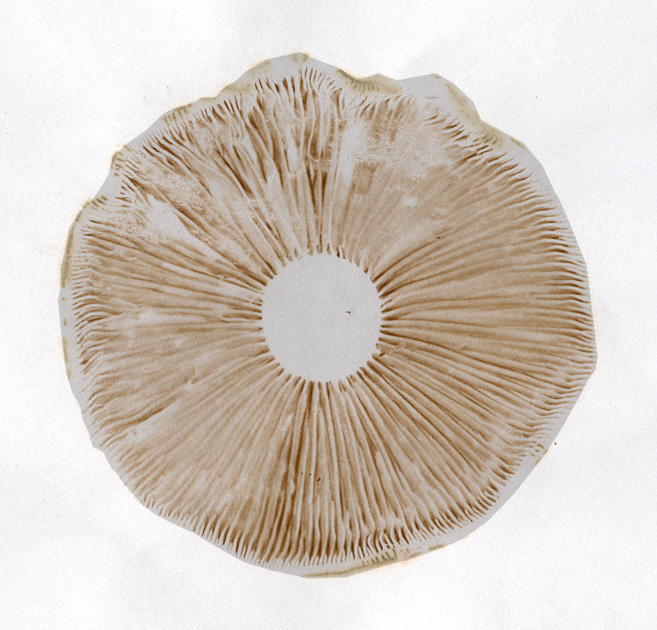In this detailed image, we're presented with a close-up view of a brownish, round structure that resembles the top or underside of a mushroom. The surface of the structure is textured with numerous light brown folds and wrinkles, giving it an irregular, spongy appearance. The circumference is notably dented, adding to the irregularity of the shape. At the center of the structure, there is a distinct circular hole with a more regular shape, suggesting the absence of the stem, typical of a mushroom. The background is a clean white, which contrasts starkly with the deep brown edges of the structure, enhancing its visibility and detail. This detailed perspective highlights the complex and natural patterns, evoking comparisons to both the form and texture of a mushroom and the delicate intricacies of marine life like fish gills.